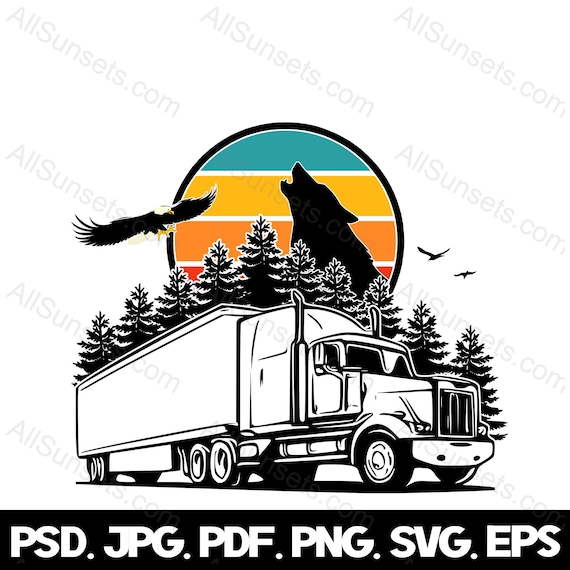This graphic features a white background with a diagonal watermark reading "allsunsets.com" across the entire image. At the bottom, a black border contains white text listing file formats: PSD, JPG, PDF, PNG, SVG, and EPS. Dominating the center of the image is a detailed black and white drawing of a large transport truck, set against a backdrop of black pine trees. Above this scene, a partially visible circle filled with horizontal stripes in turquoise, yellow, orange, and red hues encloses the silhouette of a howling wolf. To the left of the circle, an eagle with distinctive yellow beak and talons flies, while two smaller birds are depicted in black on the right side, outside the circle. The graphic appears to be a purchasable item due to the watermark's presence.